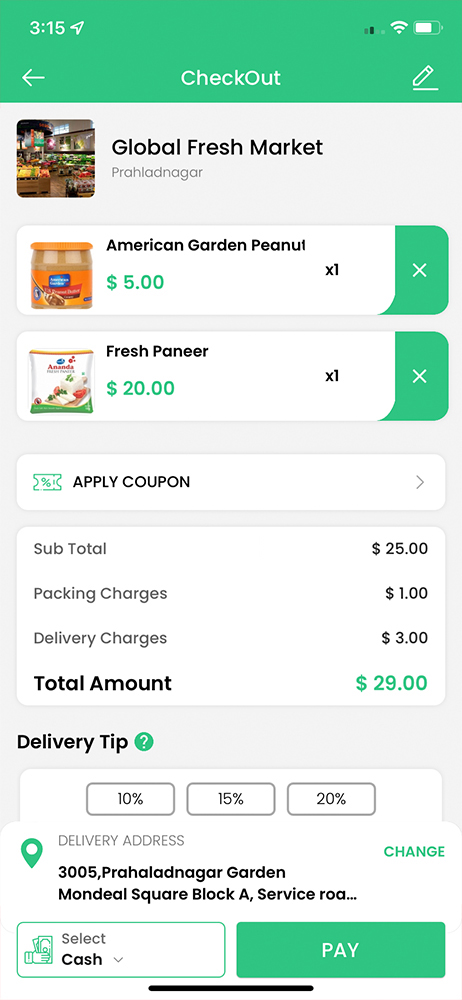This image showcases the checkout screen of an unnamed mobile app, featuring a purchase from "Global Fresh Market" located in Praldingnagar. The screen displays the details of items bought, which include "American Garden Peanut" and "Fresh Paneer," each in a quantity of one. Below the item list, there is a section indicating the applied coupon, followed by another section delineating the financial breakdown: a subtotal of $25, packing charges of $1, and delivery charges of $3, culminating in a total amount of $29. The right side of this breakdown clearly itemizes each charge. Further down the screen, there is an option to add a delivery tip with preset percentages of 10%, 15%, and 20%. Below the tip options is a section labeled "Delivery Access," and subsequently, an option for selecting the payment method. This detailed summary encapsulates all the essential elements visible in the checkout screen.